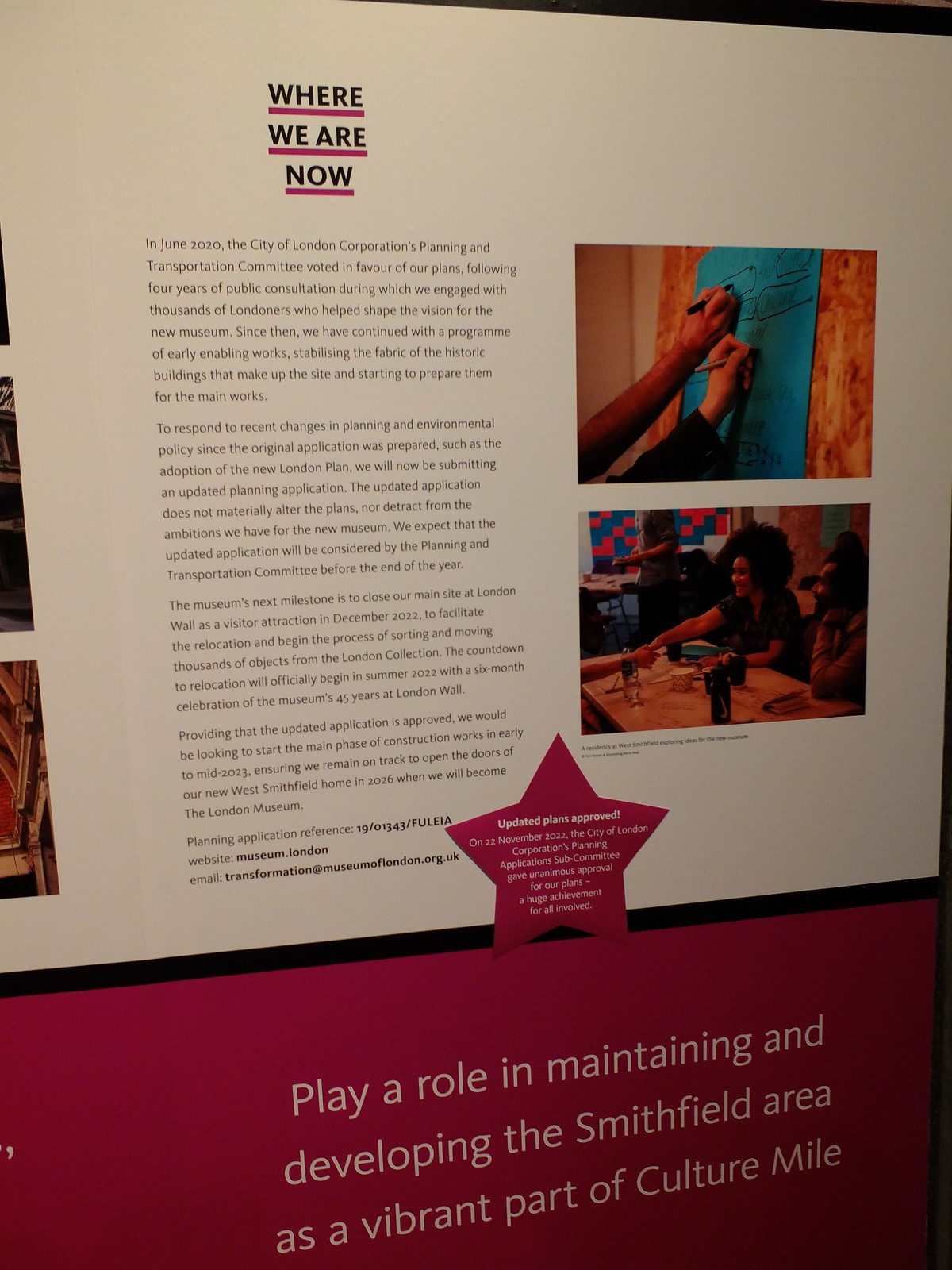This image captures a detailed display that appears to be mounted on a wall, resembling something you might see in an art museum. The prominent background is a rich magenta color, providing a striking contrast to the white and black text displayed on it. 

At the very top, the banner reads "Where We Are Now" in bold black text, underscored by a magenta line. Below this, a paragraph begins, "In June 2020, the City of London Corporation's Planning and Transportation Committee voted in favor of our plans following four years of public consultation, during which we engaged with thousands of Londoners who helped shape the vision for the new museum." Subsequent lines describe how, since then, early enabling works have stabilized the historic buildings on the site in preparation for the main construction phase. 

Further down the poster, there's a notable magenta star with white text announcing, "Updated plans approved On 22 November 2022, the City of London Corporation Planning Applications Subcommittee gave unanimous approval for our plans, a huge achievement for all involved." 

Beneath this, other sections and smaller text are present, including a call to action: "Play a role in maintaining and developing the Smithfield area as a vibrant part of Culture Mile."

Complementing the text are two notable images. The top image shows two hands writing with black ink on blue paper. Below it, another image depicts an African-American woman dining, with a glass of red wine beside her. Towards the bottom of the poster, additional paragraphs, a website, and an email address provide further context and contact information about contributions to the museum.